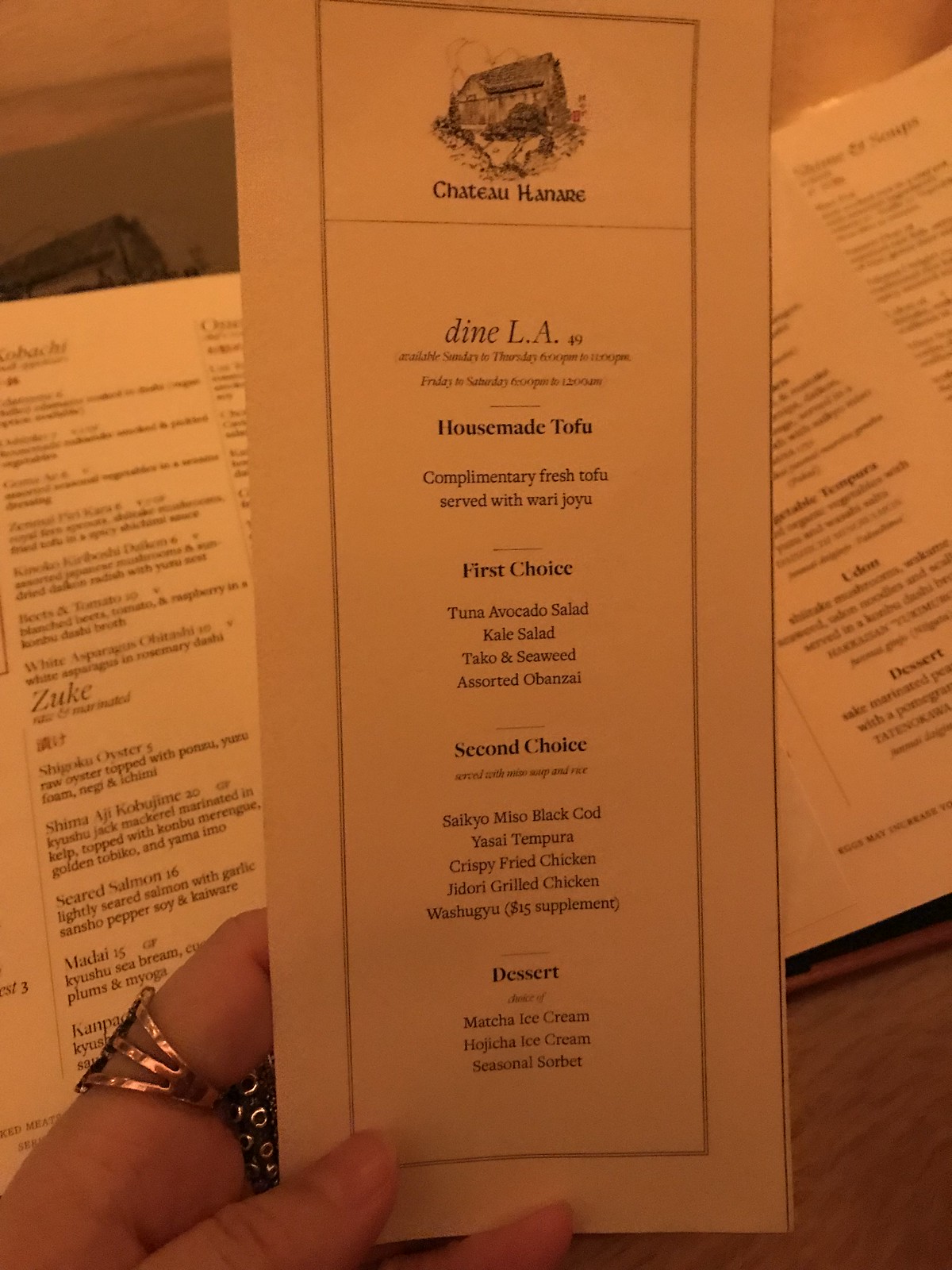In this photograph, a woman’s left hand holds a special menu for the restaurant Chateau Hannes. Her hand is adorned with two distinct silver rings: one on her index finger featuring an open tri-colored band with a shiny finish, and another on her middle finger showcasing a hammered metal design with octopus-like embellishments. The special menu she grasps is a long vertical piece of ivory paper, adorned at the top with an intricate drawing of the restaurant framed inside a box. Below the illustration, the centered black text lists various categories, including "House-Made Tofu," "First Choice," "Second Choice," and "Dessert," each accompanied by four to five unique dining options.

In the background, a regular restaurant menu lies open on the tabletop. This standard menu matches the special one in its ivory color, featuring multiple columns of text meticulously printed in black type. The background scene subtly emphasizes the detailed nature of both menus, providing a comprehensive glimpse into the dining experience at Chateau Hannes.